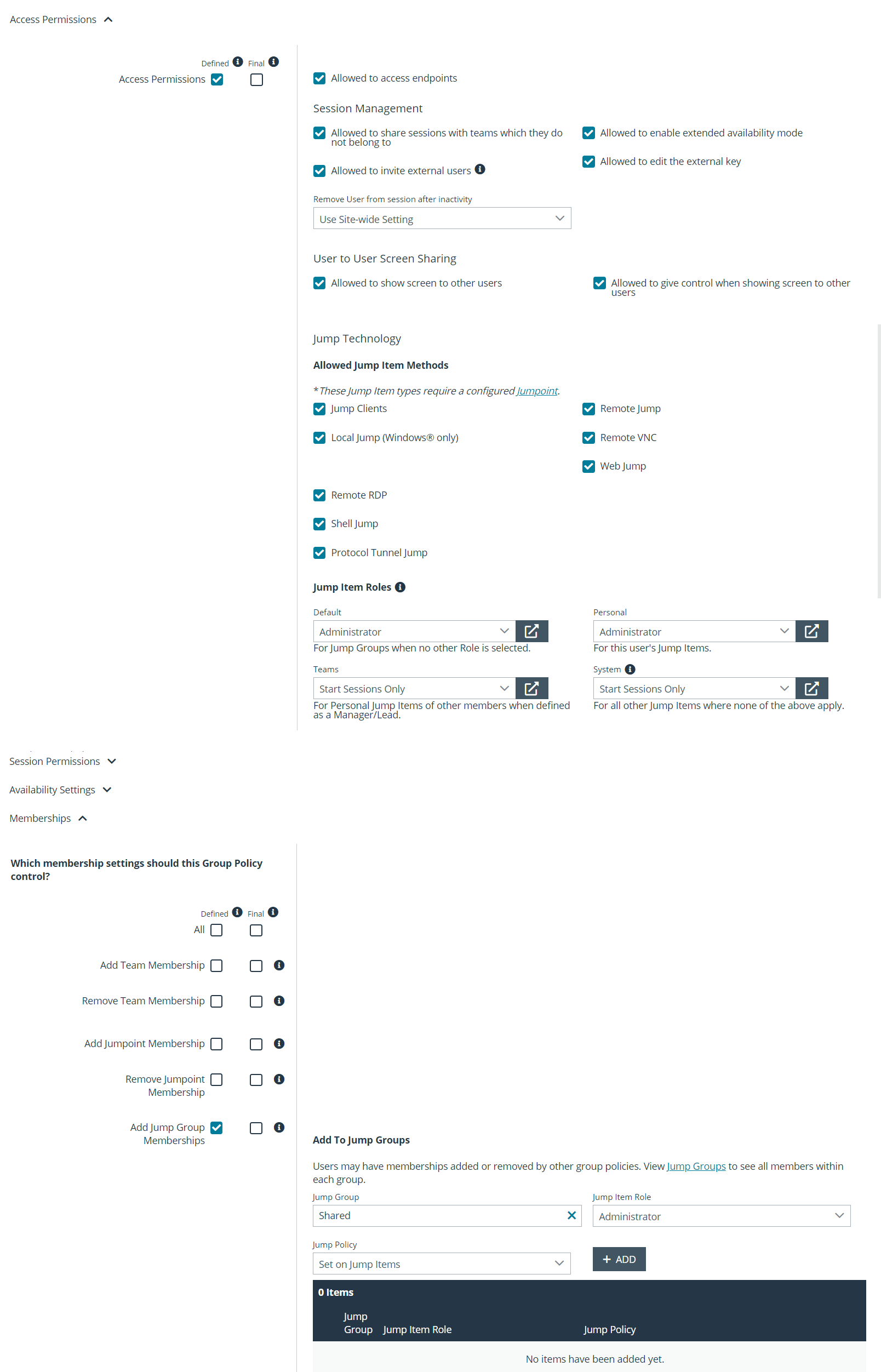This is a detailed caption for your image:

---

The screenshot depicts a website’s permissions page, clearly designed to manage and configure various access settings. The image appears quite small, necessitating enlargement for better legibility. At the top left corner, the title "Access Permissions" is prominently displayed next to an upward-pointing arrow, indicating that clicking on this arrow will reveal detailed information about this section. Below this header, there are two checkboxes labeled "Defined" and "Final," accompanied by an information icon (an eye) that offers additional explanations for these terms. The "Defined" checkbox is selected.

Further down the page, there are several sections with comprehensive lists of items, most of which are checked off. For instance, the “Jump Technology” section is fully checked, indicating all items within this category have been permitted. This includes functionalities like “User-to-User Screen Sharing” and "Session Management," both thoroughly marked.

However, not everything is enabled; the "Membership Settings" at the bottom left of the page shows unchecked items, specifically options for adding "Jump Group Memberships." This suggests that the current configuration does not include access to certain membership features, possibly indicating that the user does not possess a related membership account. 

---